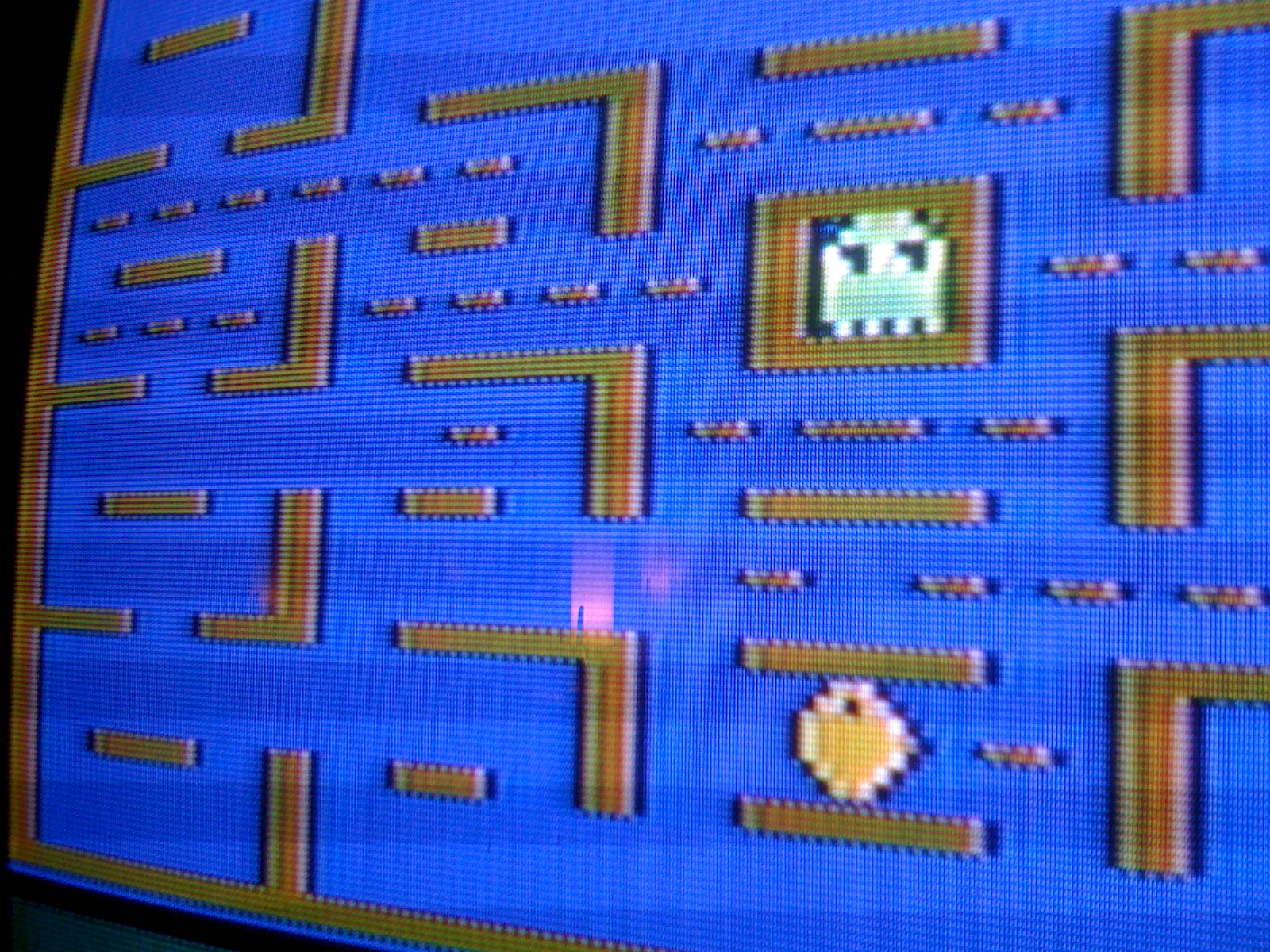This is a close-up photograph of a TV screen displaying the Atari 2600 version of Pac-Man, widely regarded as the most inferior iteration of the game when compared to the original arcade release. The image is slightly out of focus and not very sharp, revealing the curvature characteristic of older video screens built into vintage arcade machines or tabletop arcade games commonly found in bars and restaurants. The majority of the picture is dominated by the game screen, which occupies about 95% of the frame, with minimal black borders on the left edge and bottom right corner. The game's blue background consists of alternating lighter and darker blue stripes, and the playfield is filled with L-shaped boundary lines pointing in various directions. Central to the image is a brown square containing one of the 8-bit ghosts, depicted in a light gray-green color. Towards the bottom right of the screen is the yellow, 8-bit representation of Pac-Man, which, despite being designed to look round, appears significantly pixelated. The screen is devoid of any text, enhancing the authentic retro aesthetic of this broken, poorly controlled version of the iconic game.